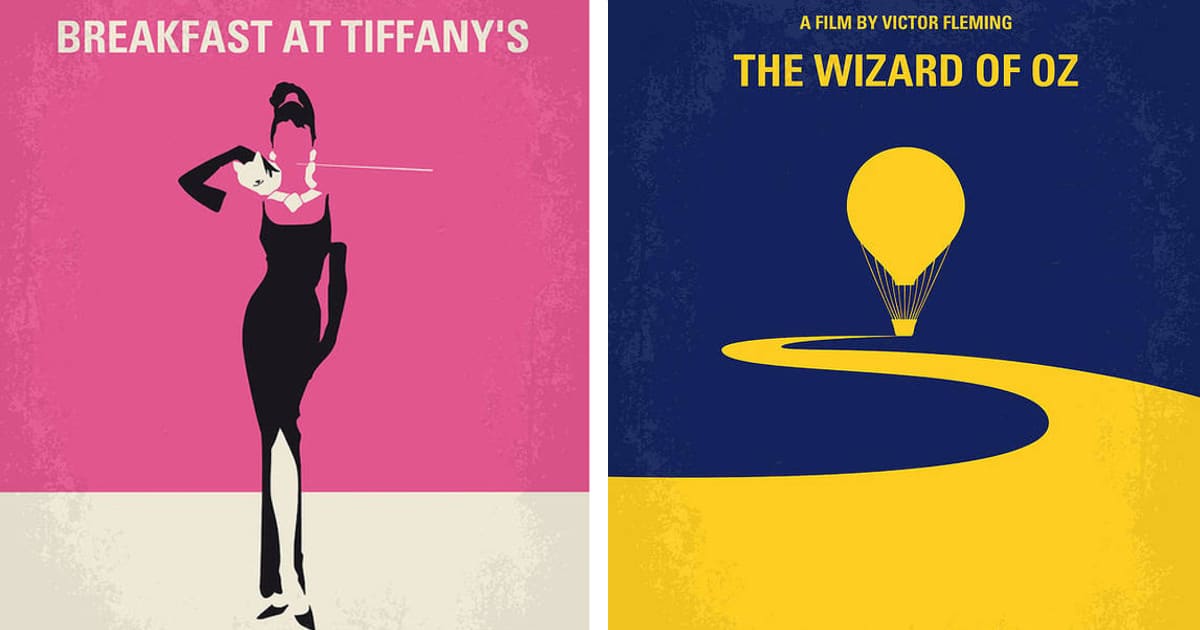The image features two side-by-side, minimalist movie posters. The left poster is for "Breakfast at Tiffany's" and has a predominantly hot pink background with a white bottom fifth. Central to the design is a silhouette of a woman, likely Audrey Hepburn, wearing a black dress with spaghetti straps, long black gloves, and pointed black shoes. Her face and exposed skin are pink, creating a stark contrast against the black of her attire. She also sports a white necklace and appears to hold a long, thin object, possibly a cigarette holder or a conductor's baton. The text "Breakfast at Tiffany's" is written in white at the top of the poster. 

The right poster, for "The Wizard of Oz," features a deep blue background with a yellow brick road snaking toward the viewer and leading to a yellow hot-air balloon. The text "A Film by Victor Fleming, The Wizard of Oz" is prominently displayed in yellow. The design is vibrant, with the blue and yellow creating a visually striking contrast. Both posters use simple color palettes and silhouettes to convey the essence of the movies.